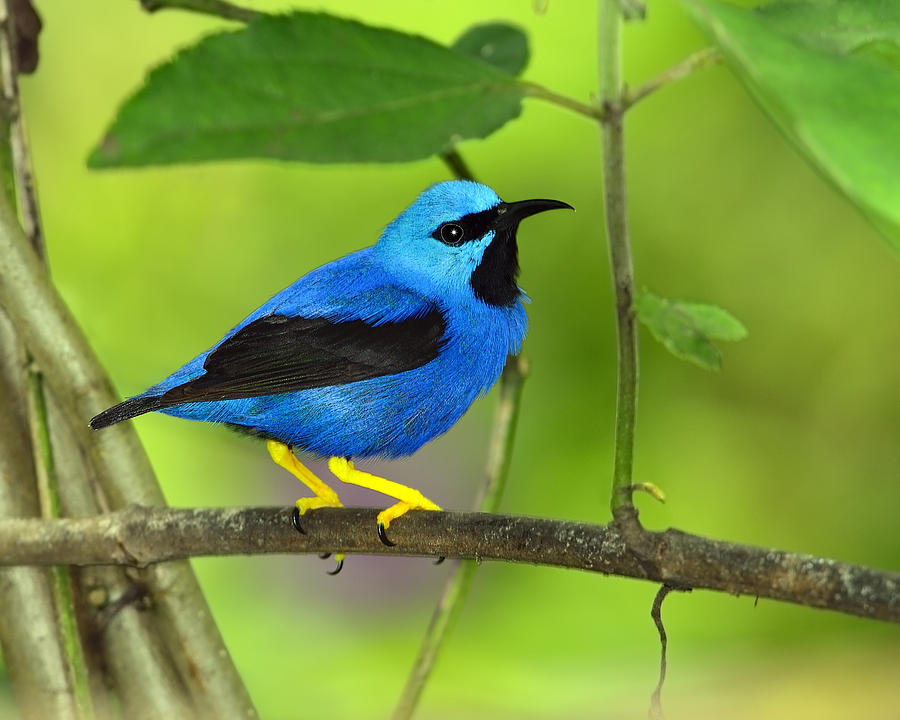The image captures a close-up of a small blue bird perched slightly to the left of center on a tree branch. The bird, facing to the right, showcases a vibrant blue head and body, with a striking black beak, black eyes, and a distinct black throat. Its wings are primarily black, with the outermost feathers also black, contrasting sharply with the blue. The bird's yellow legs and black talons grip the branch firmly, wrapping around it.

The background is artistically blurred, featuring a mix of green and subtle gray tones, drawing attention to the sharp details of the bird. Above the bird, a green leaf adds a touch of natural elegance. To the right, a smaller offshoot branch with a green leaf extends upwards, while additional branches, some leading out of the image, create a textured backdrop. This vivid nature photograph beautifully highlights the intricate details and colors of the bird amidst its natural habitat.